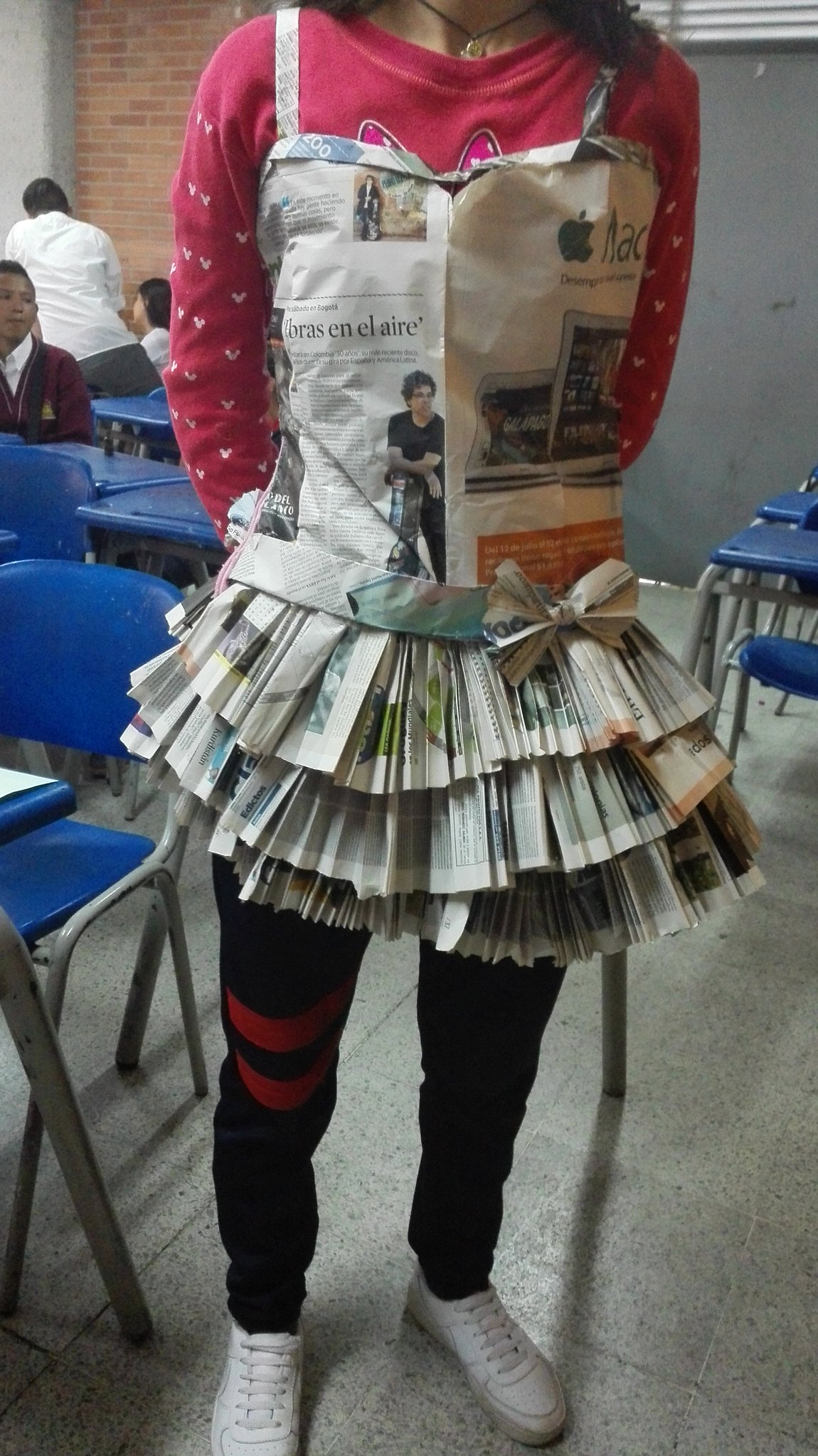In this photograph, a woman is standing in a classroom with gray tile flooring and red brick walls. Blue chair desks with silver legs are scattered around the room, and a few other people are visible in the background, sitting and facing various directions. The woman is captured from her shoes up to her neck, her face out of view. She's wearing white shoes, black capri pants or tights, and a long-sleeve shirt that is reddish-pinkish with white hearts on the sleeves.

Most notably, the woman sports a striking DIY costume—a dress made entirely of newspaper. The strapless newspaper dress features a flared skirt that ends at mid-thigh, with meticulously folded pleats forming three layered ruffles. A newspaper belt and a small bow accentuate her waist, with one newspaper strap over the shoulder. Headlines and pictures from the newspapers are visible on the dress, adding to its intricate detail. The woman stands with her arms behind her back against a backdrop of blue desks, emphasizing both her costume and the classroom setting.